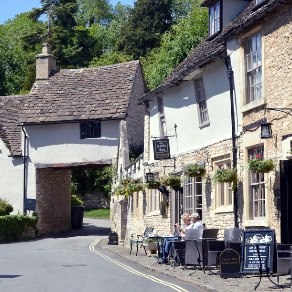The image captures a picturesque street scene in a rural village. The asphalt road emerges from the bottom left corner, flanked by a green shrub, and extends into the distance where it passes under a building with a sharp roof that arches over the street like a bridge. To the right of the street, there's a two-story stone building with multiple windows, painted white. Outside this building is a small cafe, with tables and chairs set up along a narrow sidewalk. A couple, possibly a man and a woman, sit at one of these tables, engaged in conversation. The man is wearing a hat. Above the street, a blue sky is visible, with no clouds, suggesting it's the start of the evening. The scene is enveloped by a serene grove of trees, visible along the route of the street, adding a lush green backdrop to the setting. A restaurant signboard stands out in the lower right corner, indicating the presence of the cafe. The overall atmosphere is calm and inviting, with the interplay of natural and architectural elements creating a charming village setting.